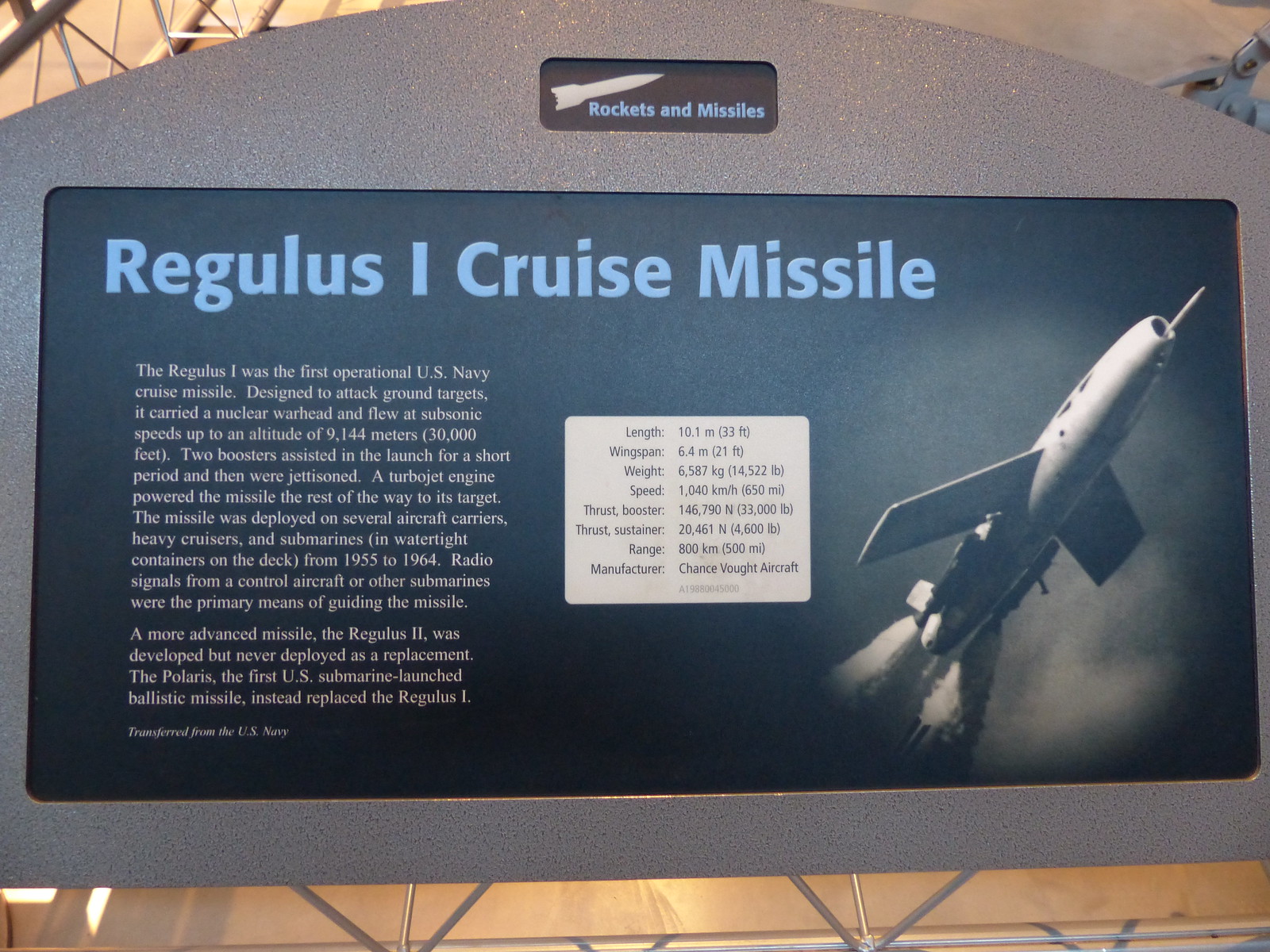The image is a color indoor photograph of a museum display showcasing information about the Regulus I cruise missile. The display, which is rectangular and bears a resemblance to a tombstone with a curved top and squared sides and bottom, is made of gray stone. At the top of the display, there's a small card featuring a drawing of a white missile, labeled "rockets and missiles." Below this card, in large blue font, is the title "Regulus I Cruise Missile."

The main body of the plaque provides detailed information about the missile:

"The Regulus I was the first operational U.S. Navy cruise missile designed to attack ground targets. It carried a nuclear warhead and flew at subsonic speeds up to an altitude of 9,144 meters (30,000 feet). Two boosters assisted in the launch for a short period before being jettisoned. A turbojet engine powered the missile the rest of the way to its target. The missile was deployed on several aircraft carriers, heavy cruisers, and submarines in watertight containers on the deck from 1955 to 1964. Radio signals from a control aircraft or other submarines were the primary means of guiding the missile. A more advanced missile, the Regulus II, was developed but never deployed as a replacement. Instead, the Polaris, the first U.S. submarine-launched ballistic missile, replaced the Regulus I."

To the right of the text is a black and white image of the Regulus I missile, which looks similar to a jet airplane with stubby wings and an open nose, flying upwards and to the right. Directly below the main text, there's a small italicized note that reads, "transferred from the U.S. Navy."

Additionally, positioned between the main text and the image of the missile, is a white box listing the missile's specifications in black text:
- **Length:** 10.1 meters (33 feet)
- **Wingspan:** 6.4 meters (21 feet)
- **Weight:** 6,587 kilograms (14,522 pounds)
- **Speed:** 1,040 kilometers per hour (650 miles per hour)
- **Thrust (Booster):** 146,790 Newtons (33,000 foot-pounds)
- **Thrust (Sustainer):** 20,461 Newtons (4,600 pounds)
- **Range:** 800 kilometers (500 miles)
- **Manufacturer:** Chance Vought Aircraft

The background of the photograph contains indistinct supporting structures such as columns and cross beams, suggesting the setting is within a larger museum or science center.